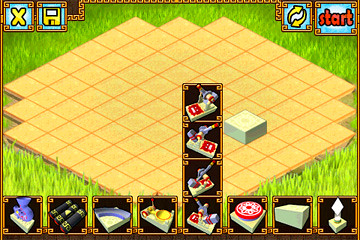This screenshot captures what appears to be a mobile game interface, likely within the tower defense genre. In the top left-hand corner, an 'X' button for closing the menu and a floppy disk icon for saving progress are clearly visible. On the top right, there is a refresh button depicted by two arrows circling each other, indicating a reset or reload function, alongside a prominent start button.

The bottom of the screen is lined with eight distinct icons, each representing various in-game items or functions. These icons are interactive, likely allowing players to tap on them to expand and explore more options or utilities. The central portion of the screen displays a grid pattern, typical of strategy or tower defense games, where different elements or units could be positioned. However, the exact details of the gameplay remain unclear from this single image. Overall, the layout and icons suggest a complex and interactive gaming experience designed for mobile platforms.